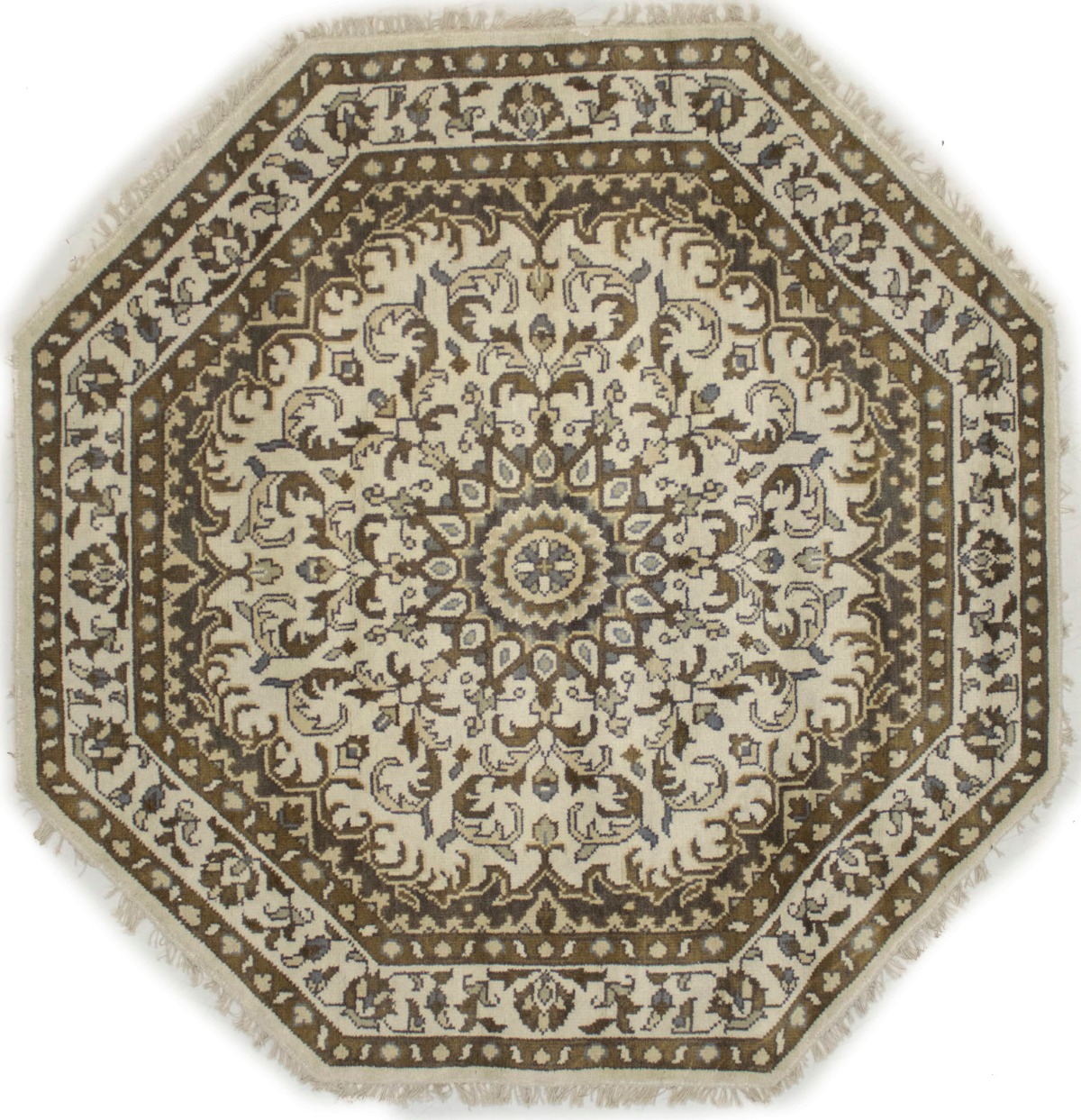The image features an intricately designed, octagonal rug with eight sides, framed by beige tassels along its border. The rug displays alternating bands of brown and tan hues that enclose a complex array of smaller, concentric circles, each adorned with floral petal motifs and additional octagonal patterns extending toward the edges. The overall palette includes cream, light blue, light green, light brown, and darker brown shades. A notable detail is the central design, which resembles an X. The rug appears to be meticulously woven, reminiscent of Persian craftsmanship, adding an elaborate and sophisticated touch to its appearance.